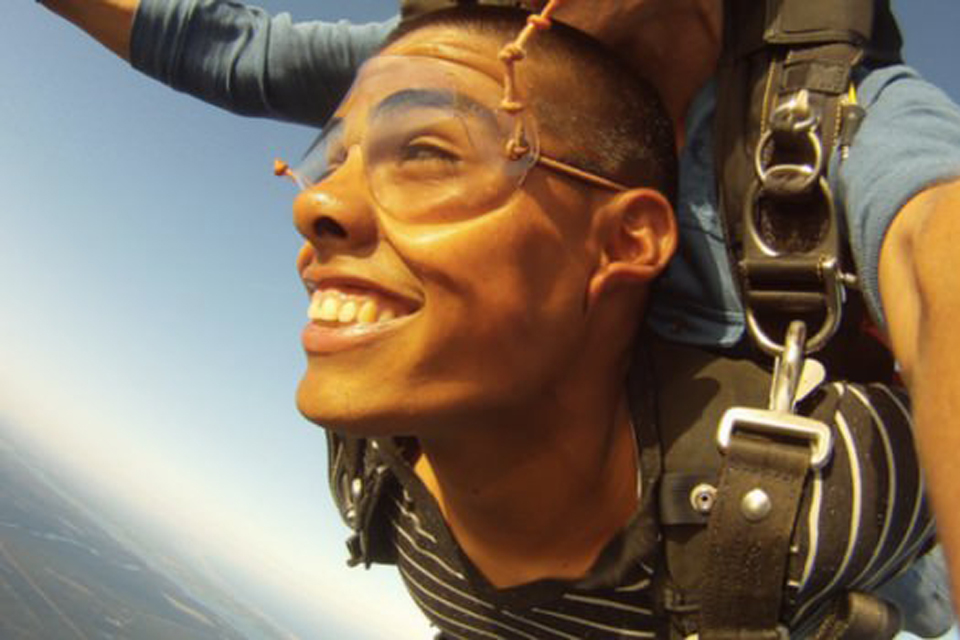This detailed photograph captures two individuals in the exhilarating act of skydiving, focusing closely on the face of the primary skydiver, who is strapped to an instructor. The main subject is a young, tan-complexioned man with almost shaved, very short black hair and a wide, joyful smile that reveals his teeth. His ecstatic expression is emphasized by the way his facial skin folds back against the wind. He is wearing snug-fitting clear goggles and a black t-shirt with horizontal white stripes. Across his shoulder runs a black strap secured by a silver buckle, attaching him safely to his tandem partner, whose blue-shirted arm and side are partially visible. The background is dominated by a vast, open sky of light blue with a gradient towards white near the horizon, along with a blurred hint of the earth or terrain visible towards the lower left of the image, emphasizing the height from which they are diving.